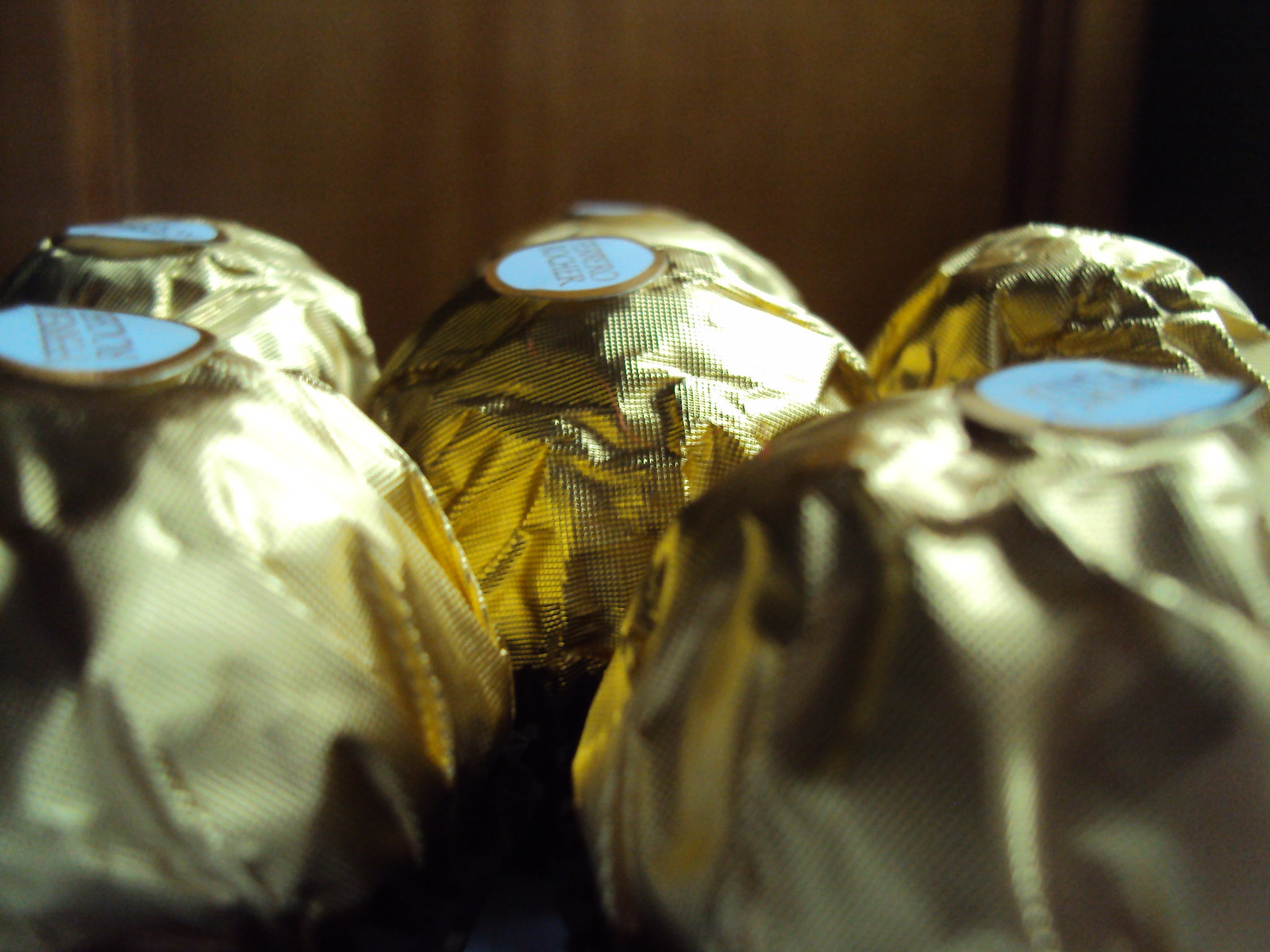This detailed close-up photograph features six Ferrero Rocher chocolate hazelnut truffles, beautifully wrapped in shiny gold foil. The candies are arranged in three columns of two, with the middle column set slightly deeper into the image, creating a sense of depth. Each truffle is adorned with a round light blue sticker outlined in dark gold, with "Ferrero Rocher" elegantly inscribed in gold lettering, except for the top right truffle which is missing its sticker. The candies take up the bottom two-thirds of the image, while the blurred brown wooden wall serves as a minimalistic background, focusing attention on the luxurious presentation of the truffles.